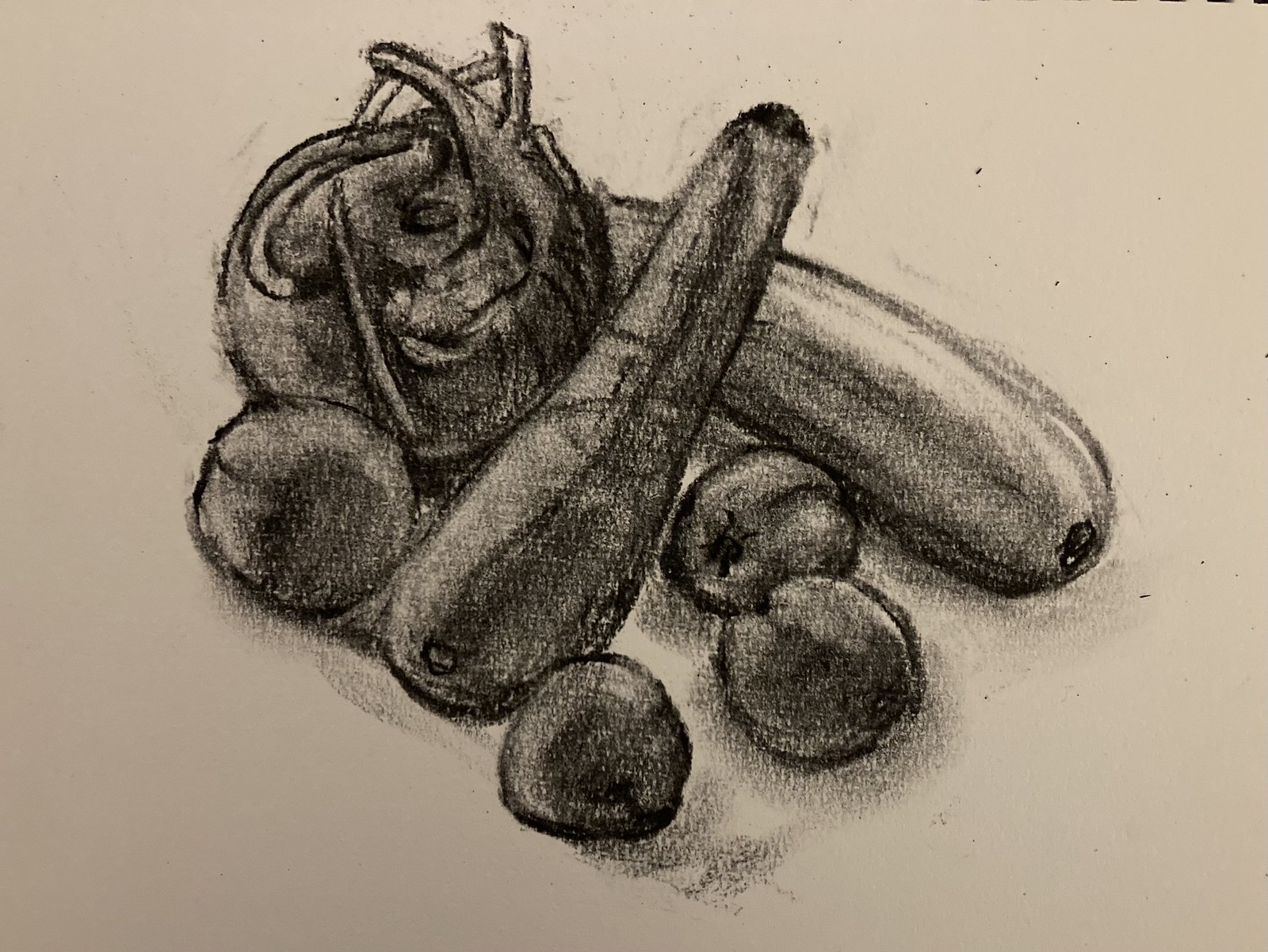This charcoal drawing on cream-colored paper features a central arrangement of various vegetables. The composition includes two elongated vegetables, one of which leans against the other. These could be interpreted as zucchini, squash, or even eggplants, rendered with significant shadowing that gives them depth. Among them, one has a distinctive black spot and a black line along its side. 

In front of these, there are four rounded vegetables, likely apples or tomatoes, given the presence of stems and their characteristic roundish shapes. Their surfaces are accentuated with light and dark gray tones to suggest texture in this black and white medium. There's also a dark, gourd-like vegetable centrally placed, characterized by varying shades from light gray on the left to dark gray and black on the right side, adding to the visual complexity.

Additionally, a partly concealed cylindrical vegetable lies among the other objects, displaying a gradation from white at the top to dark gray at the bottom. Nearby, a split-open onion is depicted, its layers peeled to reveal its interior, shaded in gray and black tones to highlight its texture and form. This rough yet intricate drawing captures the essence of these vegetables, prioritizing shape and shadow over precise detail, which lends it a unique, almost abstract quality.